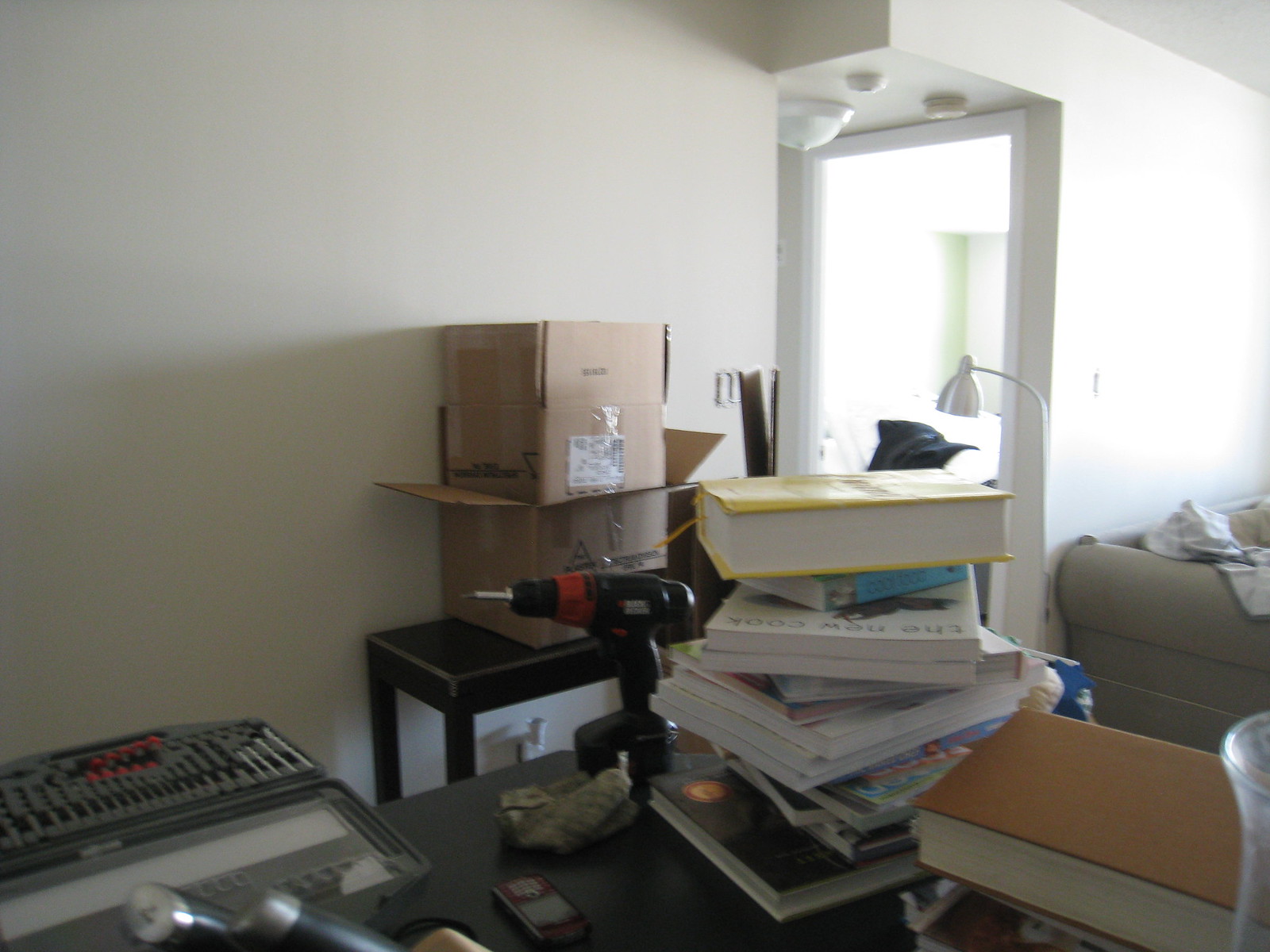The photo depicts the interior of a house or apartment with a prominent black table in the foreground, cluttered with various items. On the left-hand side of the table, there is a gray plastic toolkit, featuring multiple small compartments for different wrenches and tools, accented with some orange plastic components. In the bottom left corner, the handles of a few knives protrude from a wooden block. Also on the table is a rectangular cell phone and a towering stack of 16 books. The identifiable colors of the book covers start with yellow on top, followed by blue, white, and a brown-covered book at the bottom right corner of the stack.

A drill is also positioned on this table, contributing to the assortment of items. In the background, a smaller black table is visible, topped with several boxes. The apartment's walls are painted in a whitish eggshell hue. There is a lamp situated towards the middle right of the image, and a light-tanned couch is partially visible on the far right. An open doorway at the back leads into a brightly lit room, presumably a bathroom.